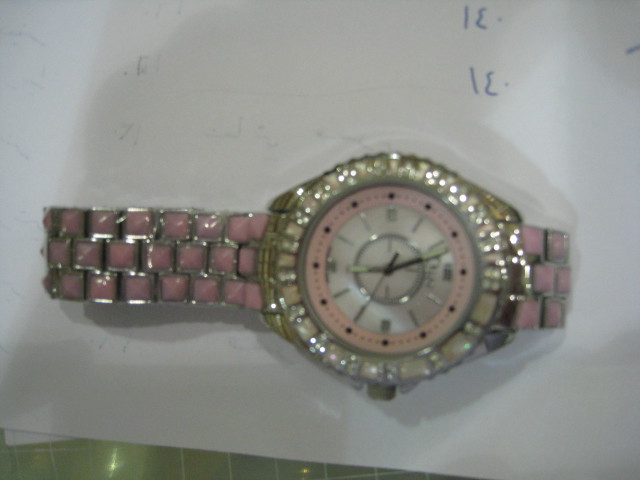A pristine white sheet of printer paper serves as the backdrop for an exquisite wristwatch. The watch boasts a circular face adorned with a dazzling array of diamonds, both across and encircling the face, adding a touch of brilliance. The face is marked by sleek silver rectangles in place of traditional numbers, showing the time as 12:26. This elegant timepiece has hour, minute, and second hands for precise timekeeping. Its strap is a standout feature, composed of three rows of pink squares that create a charming quilted effect, adding a splash of color and texture to the overall design.